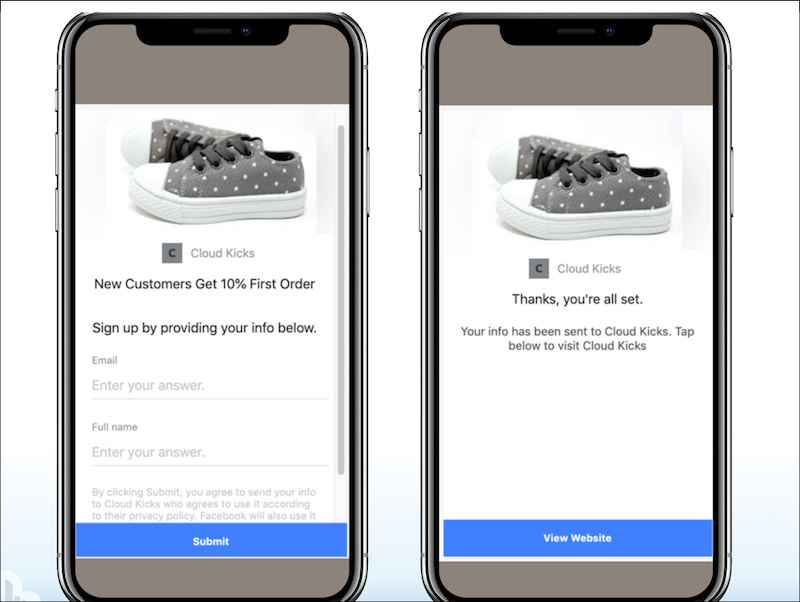The image appears to be a meticulously crafted computer mock-up featuring two identical Android mobile phones displayed side by side against a solid white background. Both phones have their screens facing forward, showcasing different stages of an online interaction with the brand "CloudKicks."

The phone on the left shows a promotional screen for CloudKicks, prominently displaying a pair of polka-dot shoes. Above the shoes, a banner reads, "New customers get 10% off their first order." Below this, there is an invitation to sign up by providing personal information, including fields for an email address and phone number. The disclaimer beneath states that by clicking "Submit," users agree to share their information with CloudKicks, which will handle it according to their privacy policy. Facebook will also have access to the information. At the bottom of the screen, a blue "Submit" button invites users to complete the sign-up process.

The phone on the right reveals the subsequent screen users see after submitting their information. It features the same image of the polka-dot shoes, with a thank-you message: "Thanks, you're all set. Your info has been sent to CloudKicks." Underneath, users are prompted to visit the CloudKicks website by tapping a blue "View Website" button.

Overall, the mock-up effectively illustrates a seamless user experience for new customers engaging with a promotional campaign on mobile devices.